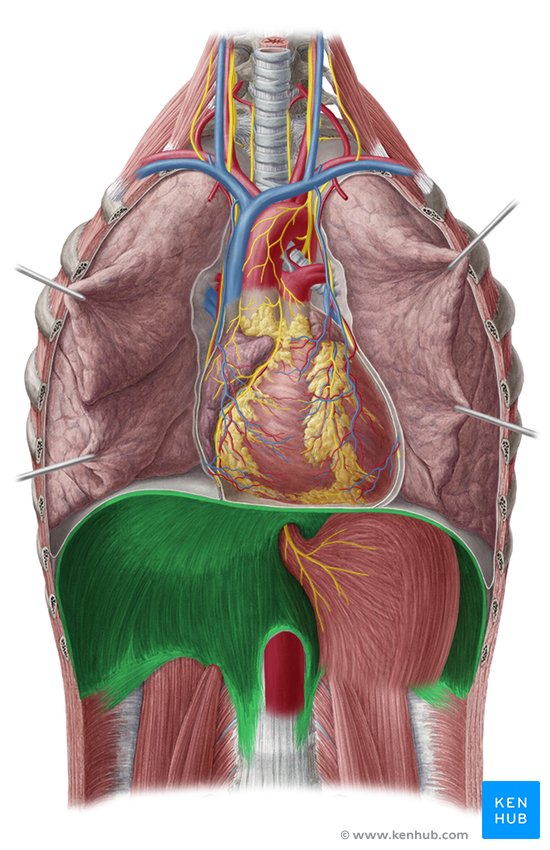This detailed illustration depicts a detailed, cutaway view of the upper human torso, focusing on the internal organs and anatomical structures. At the top of the image, we see the neck area, revealing the spine and spinal cord. The opened chest cavity is pinned back with four visible pins—two at the top and two at the bottom—exposing the organs inside. Prominently, there is a heart in the center, characterized by its pinkish color with some yellowish fat deposits. Surrounding the heart, several blue and red tubes represent the arteries and veins, along with visible nerves. Beneath the heart, there's a large green area, possibly depicting the liver or another organ, and a pinkish muscle with yellow veins at the lower portion of the image. This illustration captures the intricate details of the human anatomy, although certain proportions seem digitally distorted, suggesting it may not be a direct representation of a real human body.